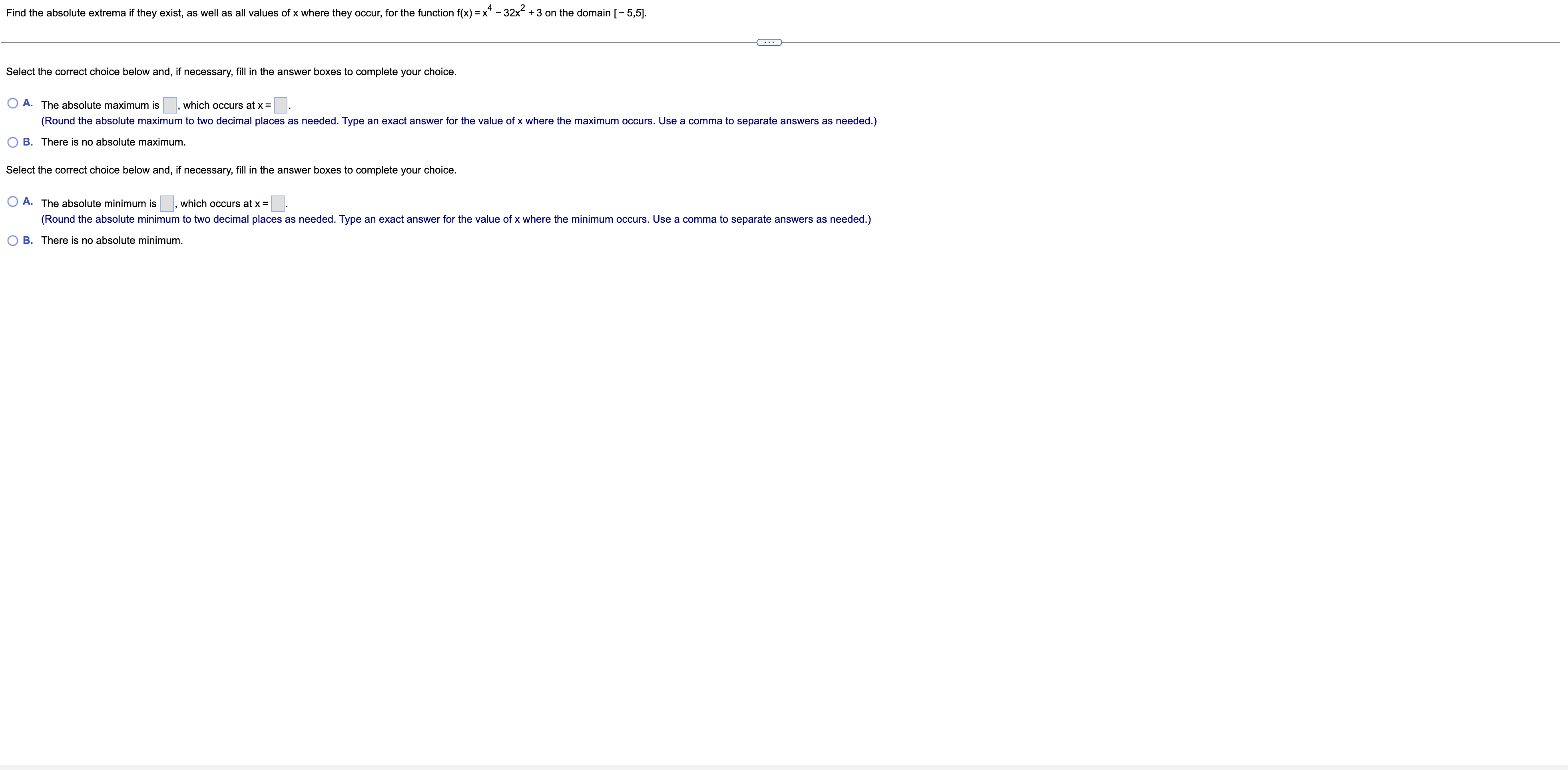In this image, we have a stark white background with very small black text positioned at the top. A thin horizontal separator line divides the content, marking a distinct break between sections. The initial line of text, which is clearly readable, is followed by blue circular icons labeled "A" and "B". Below this, another sentence appears with another pair of choices labeled "A" and "B". It seems the viewer is prompted to select the correct option if necessary, following the instruction given. Each set of choices alternates between black text and blue circular brackets around the letters 'A' and 'B', indicating required selection points for both sentences. The repetitive pattern and small font require attention to detail for accurate comprehension and selection.